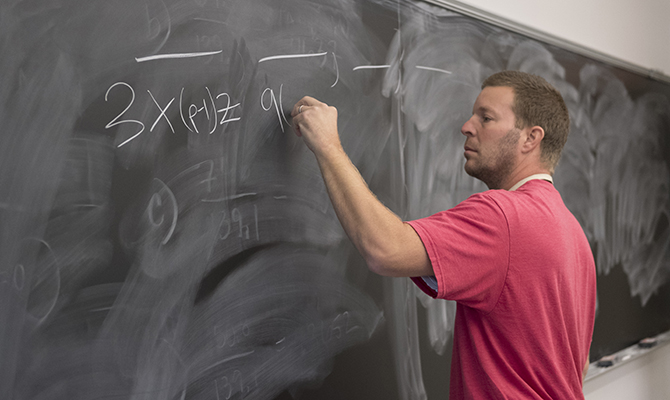The image depicts a man with short brown hair and a light stubble, possibly a teacher, standing at a well-used blackboard. He is wearing a pink shirt with a distinctive white collar, and his left hand, adorned with a wedding ring, is raised as he writes on the board with chalk. The blackboard, which dominates the photo, shows signs of heavy use, with numerous cloudy white smudge marks from previous erasures. The man is in the process of writing a mathematical equation: "3x (p - 1)", followed by either a Z or a 2, and then a 9. Additionally, parts of previously written equations like "C7", "something over 3", and "9.1" faintly show through the eraser marks. Above his writing, there are four perpendicular dashes near the top of the board. The scene suggests a classroom environment, indicative of either a student or an instructor.